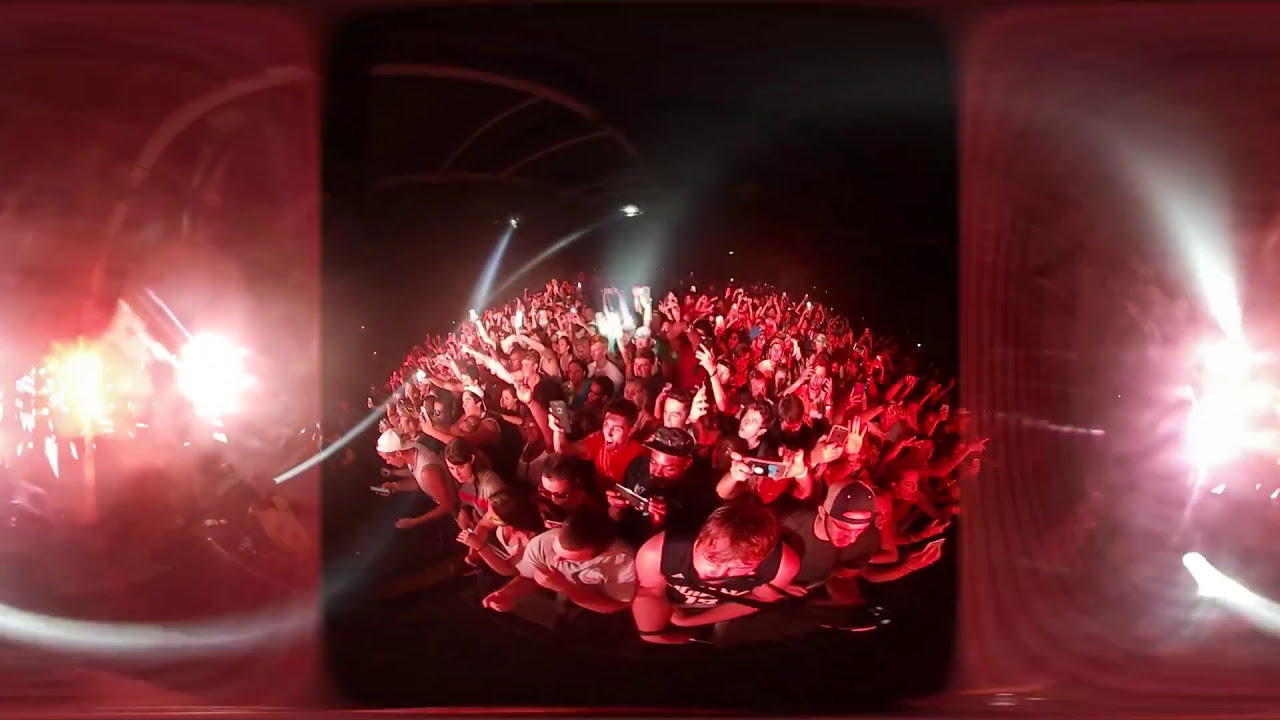The photograph captures a large, energetic crowd at an indoor concert, enveloped in a vivid red hue likely produced by the stage lighting. The image seems to use 360 imaging, creating a slightly warped appearance of the audience. Two spotlights at the top center beam down towards the stage and the crowd, illuminating the dark venue and casting a dramatic effect. The sides of the photo are blurred and blown out by intense lights, emphasizing the central mass of concertgoers. The roof's white metal support structures are barely discernible amidst the dim surroundings. In the foreground, individuals, including a man in a black sleeveless shirt with white text and another in grey, have their arms raised, some holding cell phones ready to capture the moment. Many attendees are wearing COVID masks, suggesting the photo was taken during the pandemic. The vast sea of fans extends to the back and sides, showcasing the concert's large turnout.